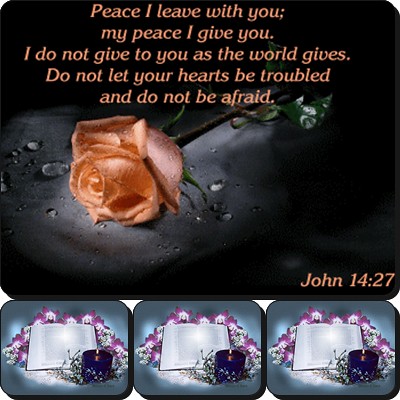The image consists of a digitally generated composition with four distinct sections. Dominating the top portion is a large, central photograph of an orange rose lying horizontally on a black surface, gradually brightening around the flower as if illuminated by a light source. The rose is adorned with glistening water droplets, and its stem and leaves are visible. Incorporated into the image is a textual overlay in a peachy-orange hue that reads, “Peace I leave with you; my peace I give to you. I do not give to you as the world gives. Do not let your hearts be troubled and do not be afraid. - John 14:27.” 

Below this main image are three smaller photographs arranged in a row. Each smaller photograph features an open book, possibly a Bible, with a lit purple candle positioned to the left. The purple candle is encircled by delicate lavender and white floral decorations. The consistent religious and serene themes, coupled with the textual message, evoke a sense of peace and spiritual reflection.